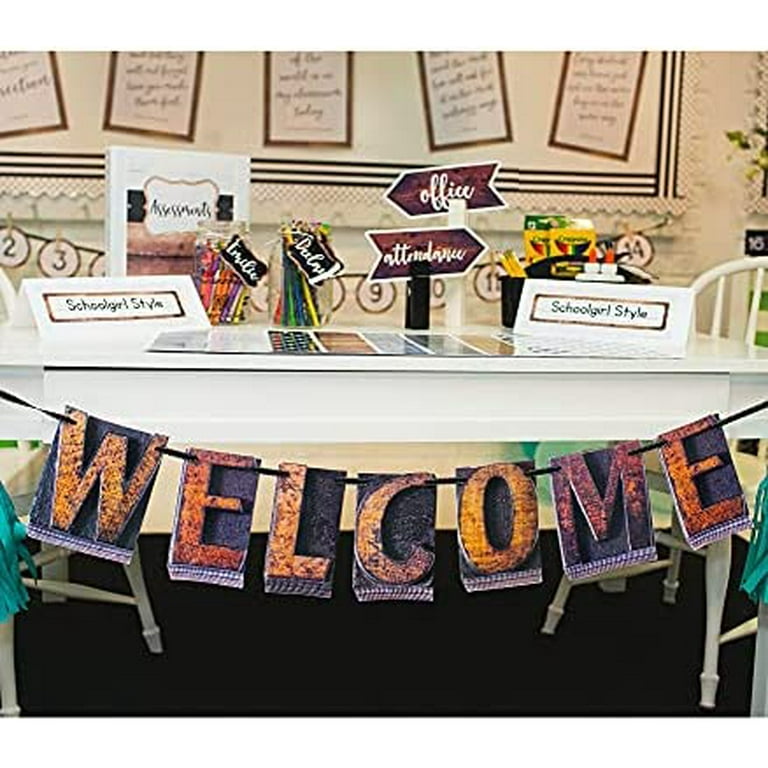This close-up photo showcases a well-decorated, rectangular white table set up for a school open house. A large welcome banner, with individual black squares adorned with orange and light orange letters, hangs across the front of the table. At both ends of the table, place cards bearing the phrase "schoolgirl style" can be seen.

On the table, informational pamphlets are neatly fanned out at the front, while two directional arrows in the middle indicate "attendance" to the right and "office" to the left. Two glass jars filled with pencils and crayons add a splash of color to the arrangement. Partially visible on opposite sides of the table are two white chairs.

The background features a black-trimmed bulletin board covered in various sheets of paper with brown backgrounds, enhancing the scholastic atmosphere. Below the table, a brown carpet completes the setting, further grounding the educational environment.